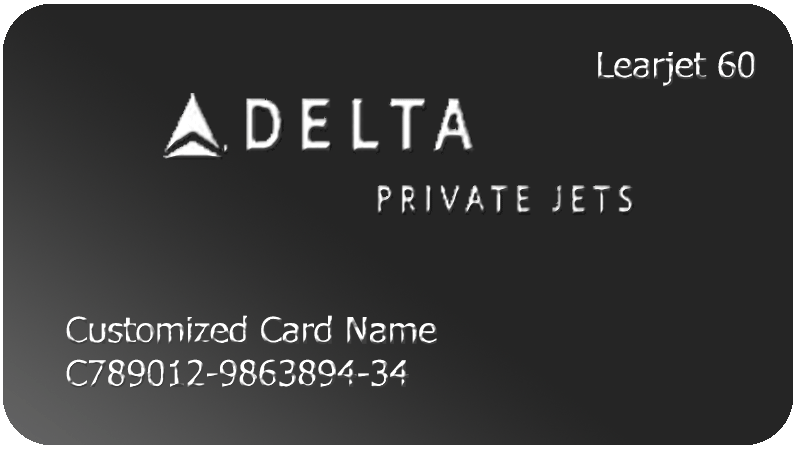This image depicts a mock-up of a Delta Private Jets card, which is designed to resemble a credit card. The card has a sleek, black background with a subtle gradient, and its edges are rounded, giving it a rectangular shape. Prominently displayed in the upper center area is the white Delta logo, consisting of a triangle atop a smaller, truncated triangle, with the word "DELTA" in all caps beneath it. Below this logo, the text "Private Jets" is also in white but is stylized to stand out in a casted character format. 

In the lower left corner of the card, there is placeholder text "Customized Card Name," followed by a sequence that appears to be a mock serial number: C789012-9863894-34. In the upper right corner, the card displays the text "Learjet 60" in silver lettering, adding to the card's premium appearance. The entire design is uniform in tone, primarily featuring shades of black, white, and silver, and lacks sharp rendering, suggesting that it is a preliminary mock-up rather than a final product.